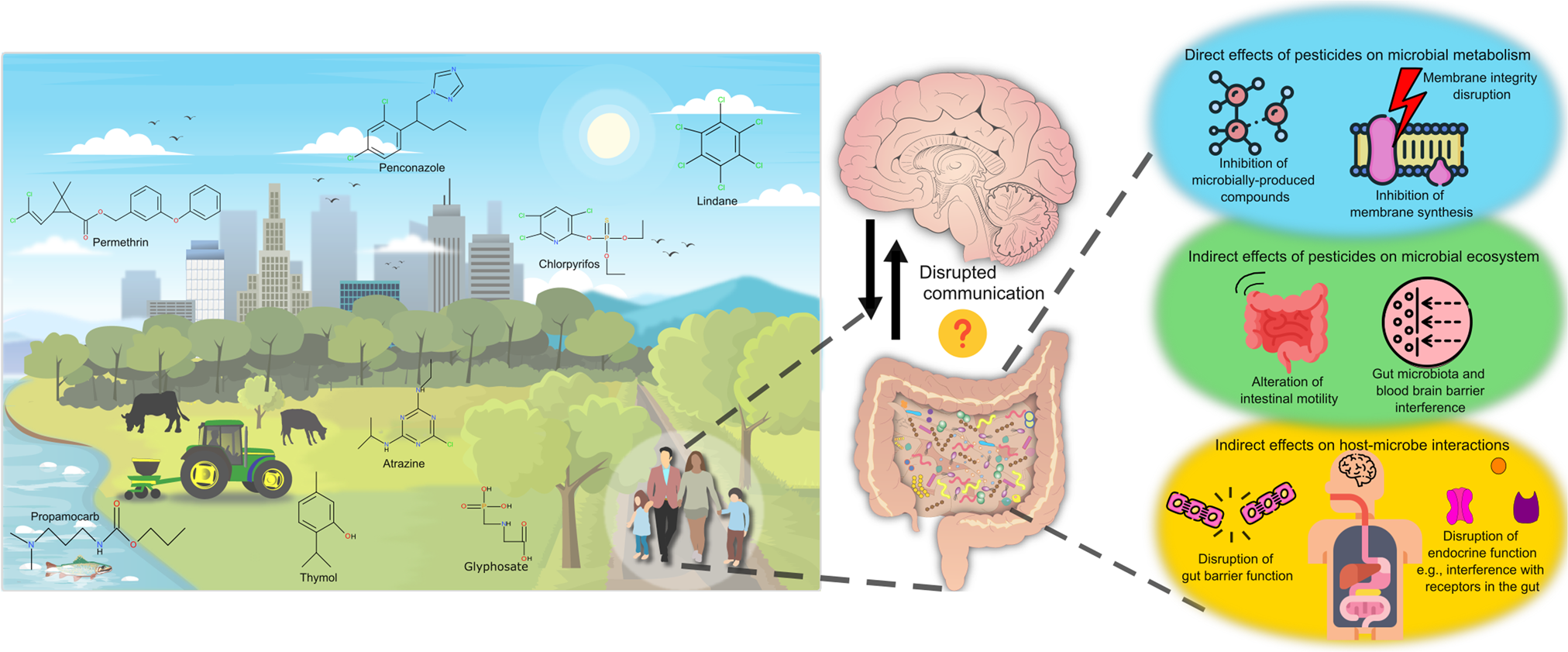The image is a detailed diagram illustrating the effects of pesticides on the human brain and body. It is divided into three distinct sections. 

The top section features a picturesque landscape with a bright sky, sun, clouds, a distant city, towering mountains, and a field with cows. Below, a diverse family of four—comprising a dark-skinned woman, a light-skinned man, and two children with mixed skin tones—strolls along a pathway. Nearby, a green tractor with yellow tires pulls a spreader dispersing pesticides and fertilizers.

In the middle section, various molecules are prominently displayed, including permethrin, penconazole, chlorpyrifos, lindane, atrazine, thymol, propamacarb, and glyphosate. Surrounding these molecules are elements symbolizing their presence in the ground and air, seemingly drifting toward the family. This section also includes detailed illustrations of the human brain with labels highlighting "disrupted communication" and "direct effects of pesticides on microbial metabolism."

The bottom section elaborates on the biological mechanisms affected by pesticides, showing diagrams of the brain and gastrointestinal system. It details the "disrupted communication" between these systems and elaborates on various direct and indirect effects, such as microbial metabolism disruption, membrane integrity and synthesis inhibition, interference with the blood-brain barrier, alterations in intestinal motility, and endocrine disturbances.

Overall, the illustration provides a comprehensive depiction of the environmental presence of pesticides and their potential impact on human health.